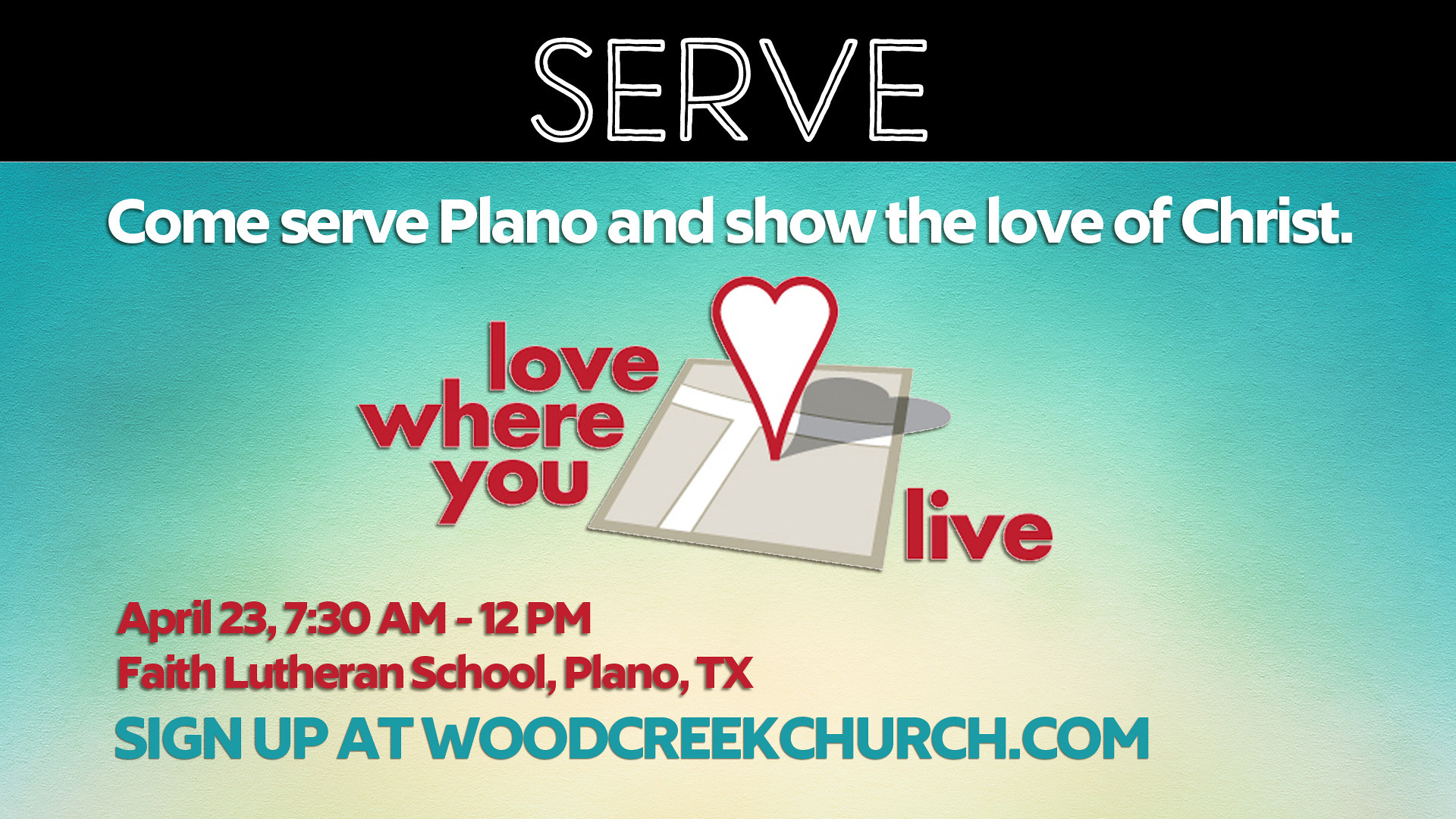The image appears to be an advertisement for a church community event, designed with a horizontal rectangular layout. At the top, there is a prominent black banner featuring the word "Serve" in a thin black stencil font outlined in white. Below this banner, the background transitions from a gradient of light turquoise blue to tan. Across this gradient, white text with a gray drop shadow reads: "Come serve Plano and show the love of Christ."

Central to the image is a map-like illustration where a white heart outlined in red marks a location, instead of a typical location pin. Flanking this heart, red text on either side reads "Love where you live." Further below, additional red text announces the event details: "April 23rd, 7:30 a.m. to 12 p.m." followed by the venue "Faith Lutheran School, Plano, Texas." The bottom part of the advertisement features blue text directing viewers to "Sign up at woodcreekchurch.com," positioned on the light turquoise and tan gradient.